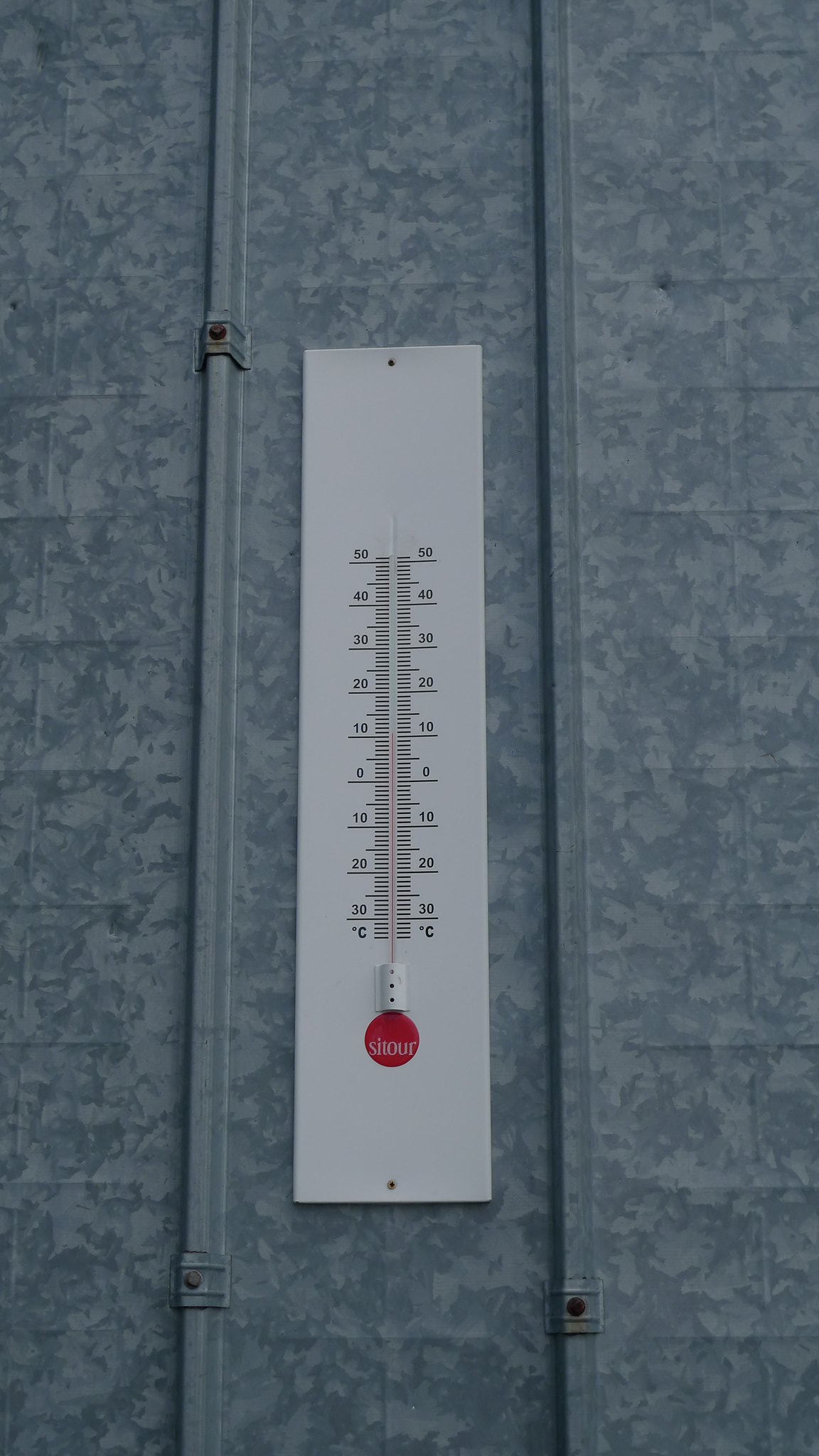The image showcases a white, elongated triangular thermometer affixed to a galvanized metal surface. The thermometer features two vertical scales, each marked in Celsius, ranging from 30 to 50 degrees Celsius. The numeral scales are accompanied by black lines for precise temperature readings. Positioned at the bottom of the thermometer is a red dot encased with the white letters "S-I-O-U-R." Above this section, there's a small white reservoir with three black dots, likely indicating the area where mercury collects.

The thermometer is secured to the metal surface by small holes located at both the top and bottom, presumably for screws. The galvanized metal background exhibits a mix of light and dark gray hues in a random pattern, contributing to an industrial texture. Additionally, the background features vertical ridges on either side, creating a bordered effect. A visible brace, held by rusted screws, supports one of the top ridges against the wall. Similar braces with rusted screws are noted at both the top and bottom edges of the surface, ensuring stability. The thermometer itself has considerable plain white areas at both top and bottom, contrasting with the detailed central scale.